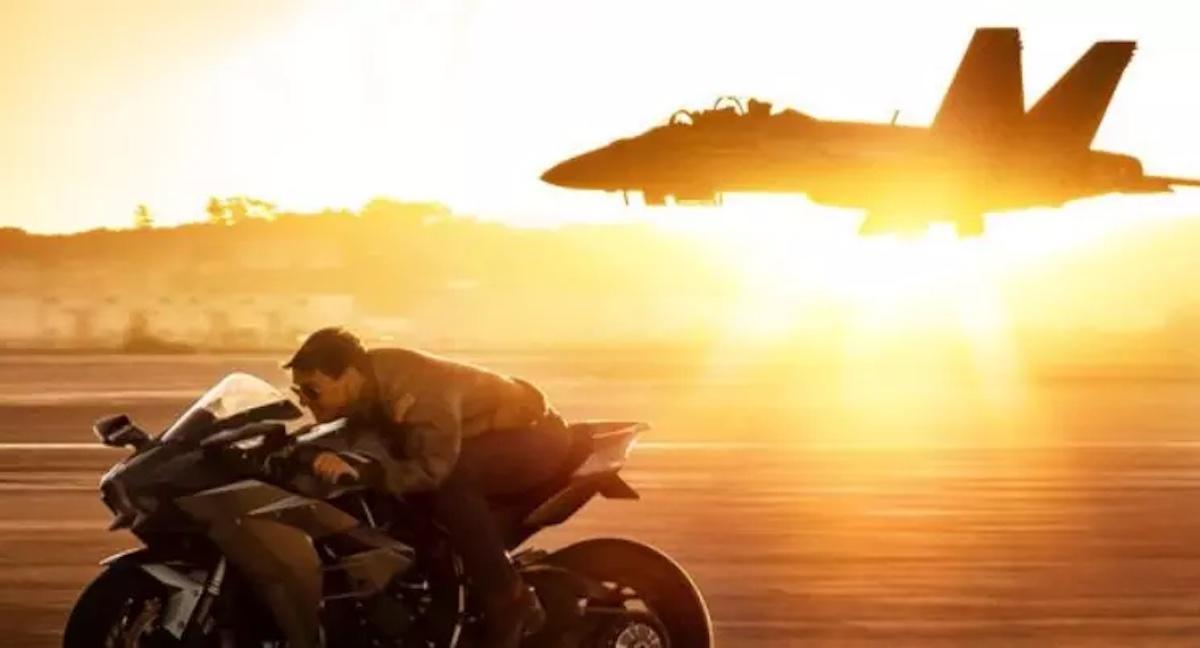The image is a low-resolution screen grab from the original "Top Gun" movie. It captures an action-packed moment featuring Tom Cruise on a sleek, black sports motorcycle, leaning low behind the windshield for aerodynamics. He dons a jacket and aviator sunglasses, speeding down a runway heading left. Behind him, an F-14 fighter jet, the same kind he flies in the movie, has just taken off, its silhouette framed against the setting sun, which bathes the scene in a vivid yellow light. The runway appears blurred, emphasizing the high speed at which both the motorcycle and fighter jet are traveling. The composition places Tom Cruise on the lower left of the image and the ascending F-14 on the upper right, creating a dynamic, high-energy snapshot from the film.